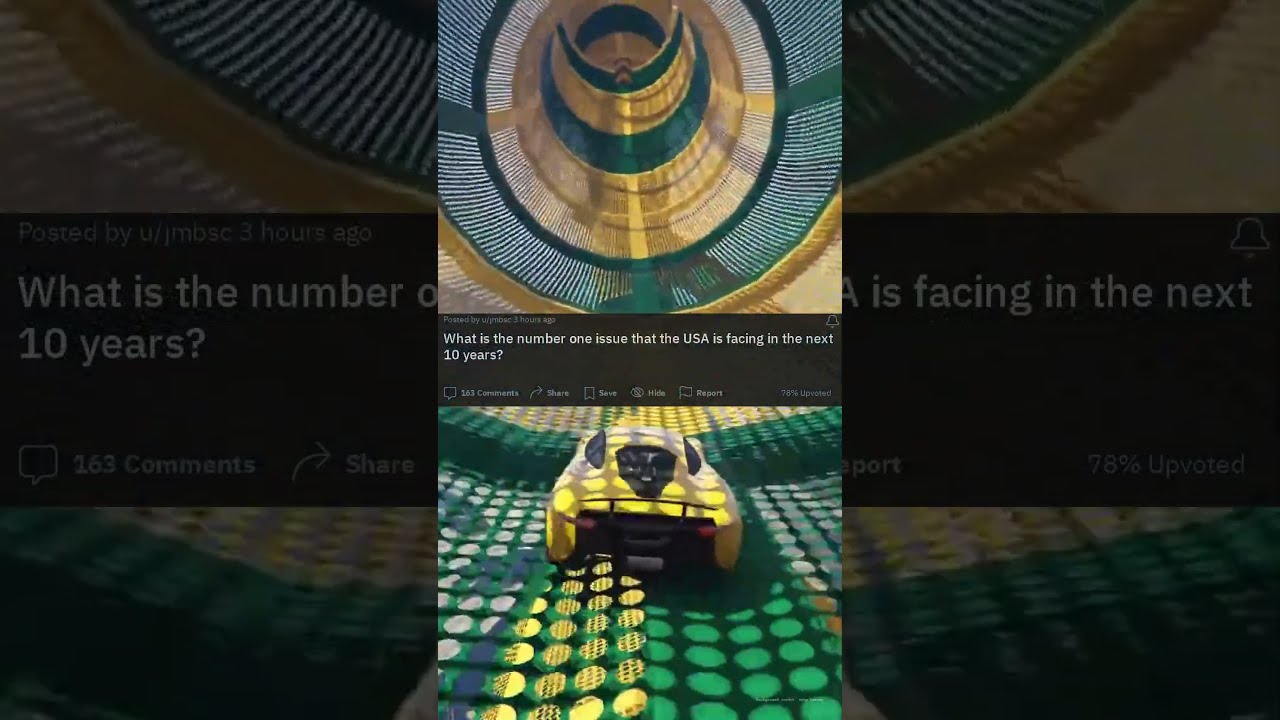The image is a color photograph that appears to be a screenshot or app display on a cell phone, presented in portrait orientation. The central image shows a futuristic yellow race car zooming down a tubular tunnel made of red and yellow netting, amidst a background of green and yellow circular patterns. The backdrop and surrounding portions of the image, displayed in darker tones and in landscape orientation, are magnified sections of the same photograph. The scene has a surreal and illustrative style, blending photographic and fantastical elements. In the central panel, a black banner with white text reads, "What is the number one issue that the USA is facing in the next 10 years?" Below this banner are icons for comments, share, save, and report, with statistics showing 163 comments and a 78% approval rate. The intricate details and layering underscore the complexity and possibly symbolic nature of the composition, hinting at an article or discussion possibly related to societal or futuristic themes.